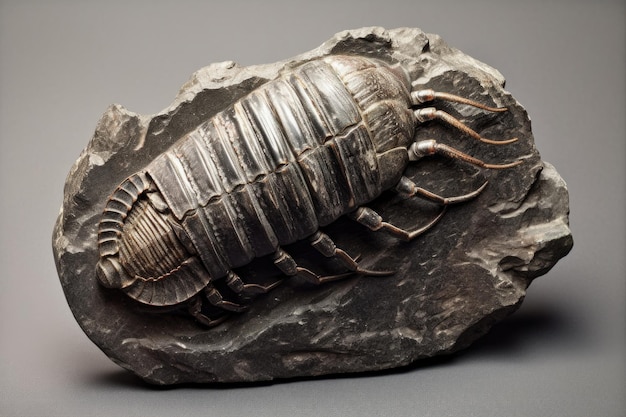A detailed description of the image:

The image features a dark gray, rugged rock that appears to be a fossil. The rock's surface is uneven, with jagged edges on the top, bottom, and sides, indicating it has not been smoothed over time. Embedded in the center of this rock is an intriguing fossilized specimen that resembles a hybrid of a beetle and a centipede or millipede. The upper part of the fossil has a hard shell characteristic of a beetle, while the right side shows multiple small legs, reminiscent of a centipede or millipede. The left side of the fossil is obscured or possibly broken, making it difficult to determine its full structure. The rock itself is displayed against a solid gray background, emphasizing the contrast and details of the fossil embedded within it.